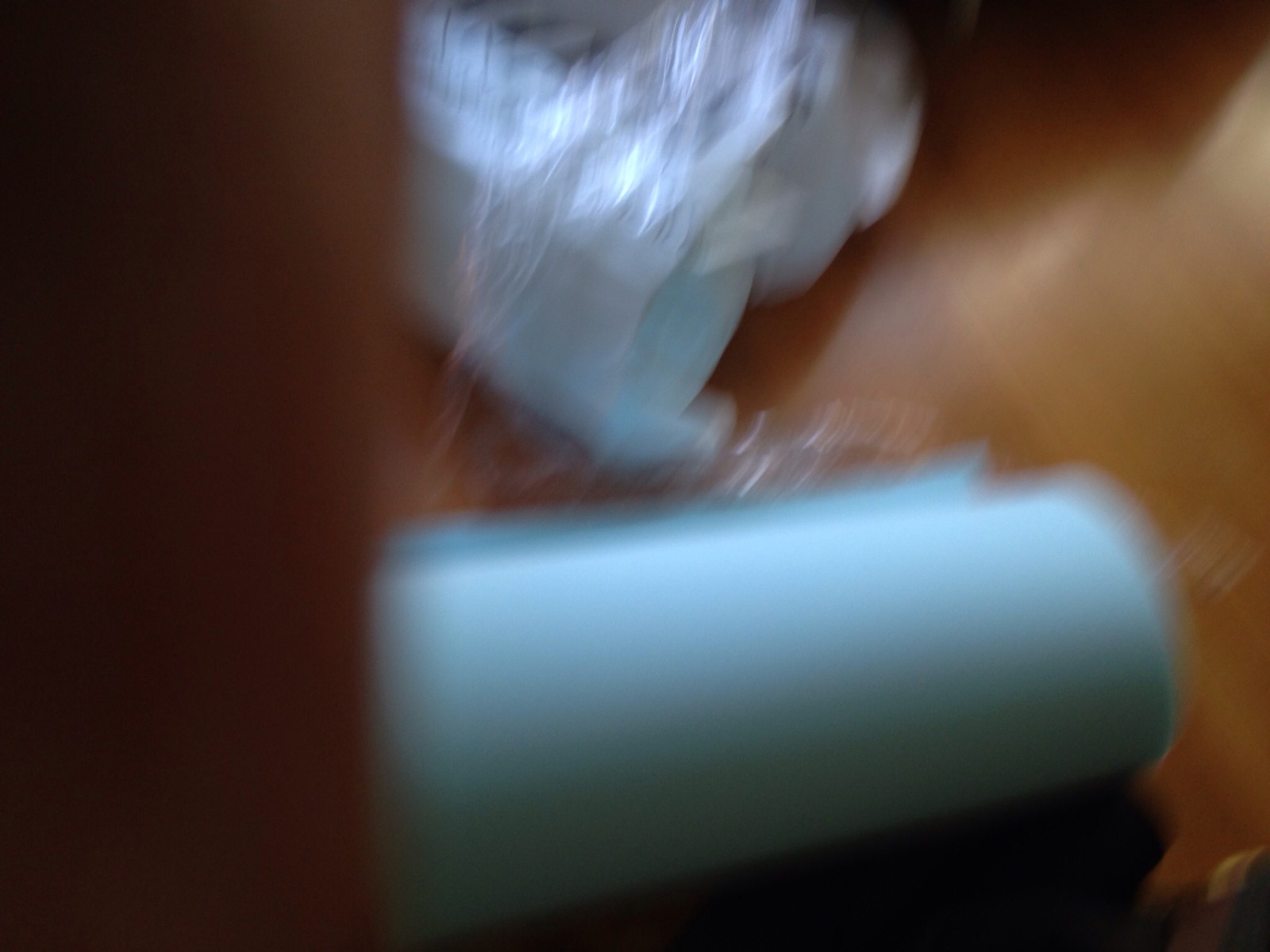A blurry photograph captures a disorganized scene on a wooden floor with a yellowish tone reminiscent of the 1970s or 1980s. In the center, a roll of blue paper towels, often associated with mechanics, is casually tossed alongside some paper or plastic wrapping, possibly from a package or the same paper towels. The upper portion of the image reveals light filtering in from a window, partially obscured by an object that might be a counter, which truncates the view on the left. The overall setting is cluttered and indistinct, with minimal details beyond the scattered items and vintage-style flooring.